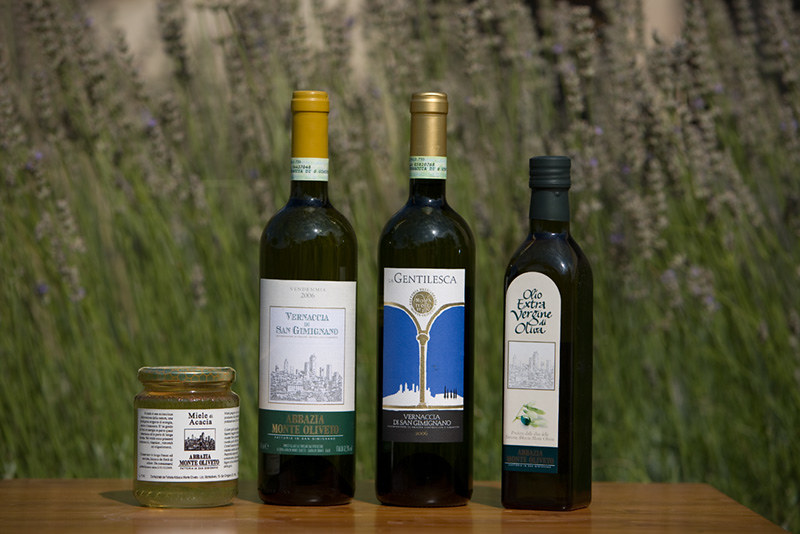In the color photograph, a dark wooden table with a high gloss finish stretches across the foreground. Set upon it are three bottles and a jar, each meticulously detailed. The leftmost item is a clear glass jar of honey, capped with a gold lid and labeled "Miel de Acacia," though most of the text is obscured. Next to the jar is a dark glass bottle of wine, crowned with a dark golden-yellow cap, its label displaying the year 2006 and words like "Vernaccia San Gimignano." The third item is another wine bottle, featuring a blue, white, and gold label with the name "Gentilesca" prominently printed. The far-right item is a bottle of olive oil, characterized by its slightly squared-off dark glass design and a label marked "Oleo Extra Virgin de Olive," complete with an olive graphic at the bottom. This elegant arrangement of items sits against a blurred background filled with tall, green stems topped with what appears to be sprigs of lavender or lupine, evoking a serene and rustic atmosphere.